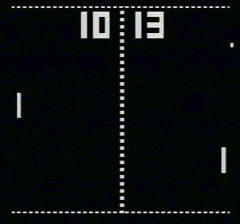This image appears to be a screenshot of an old-school video game, reminiscent of early 1980s digital table tennis, like Pong. The image is predominantly black, with white pixelated elements. A dotted white line of larger pixels runs vertically down the center, splitting the image into two halves. Additional dotted lines are visible along the top and bottom edges. On the left half, the number "10" is displayed in the upper right corner, while the number "13" is situated in the upper left corner of the right half, both rendered in retro, straight-line graphics. Two vertical white lines serve as paddles; one is centered on the left side and the other is positioned toward the bottom on the right side. Near the top right corner of the image, just below the score "13," a small white dot, likely representing the ball, is almost at the edge of the screen. This detailed setup suggests a classic competitive gameplay scene where one player leads with a score of 13 to 10.